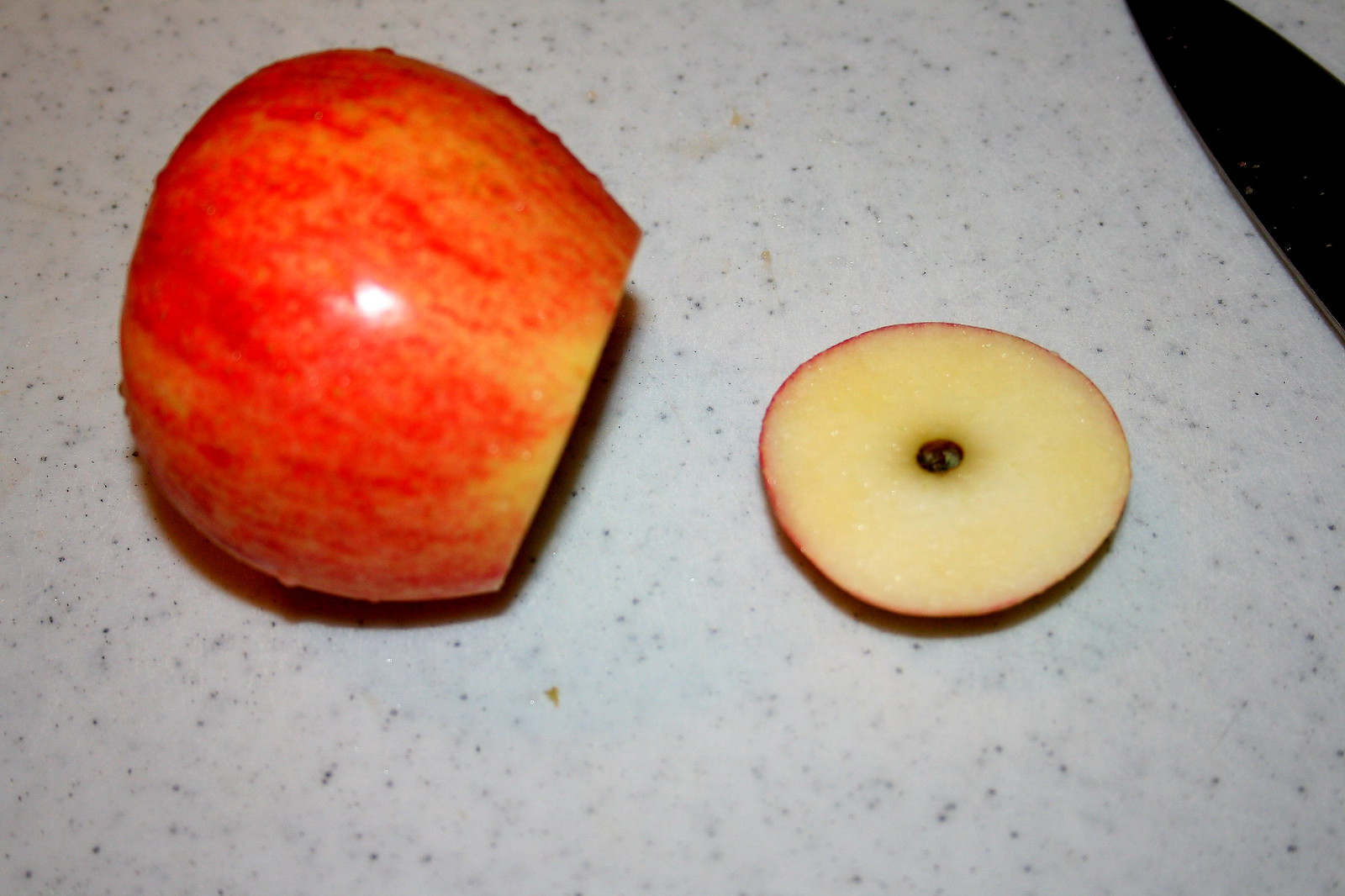A close-up image showcases a vividly colored apple sliced open and resting on a white table speckled with black flecks. The composition draws the eye predominantly to the focal point—the apple. The apple, primarily red with patches of orangish-yellow, lies on its side with a cleanly cut slice removed from the top, placed to the apple's right. The exposed core is visible and has a distinct black coloration. There are subtle shadows cast by the apple and the slice, imparting a sense of depth, while gentle light illuminates the left side of the remaining intact portion of the fruit. At the top right corner of the image, a narrow black streak adds contrast to the predominantly white table, lending a dynamic edge to the scene.